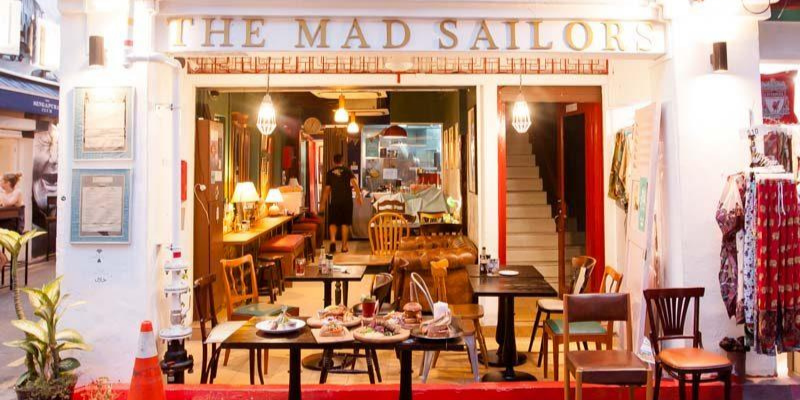The image showcases the Mad Sailor's Cafe, an inviting outdoor restaurant. Dominating the top center, a sign in gold block letters on a white background proudly displays the cafe's name. In the foreground, a vibrant red curbside table is laden with various food items, including what might be burgers and a glass of iced tea, surrounded by several chairs. On the left, a plant and an orange traffic cone add a touch of color and safety. The patio seamlessly opens into the main room of the cafe, visible through the middle of the image. Inside, lamps on several dark tables illuminate the space, where a man dressed in black shorts and a black t-shirt can be seen. The left wall features two framed menus, adding to the cafe's charm. To the right, a red doorway with white stairs leads to the second floor, complete with a light above the entrance. The setting is brimming with warm colors - shades of white, brown, red, and tan - contributing to the cozy atmosphere of the well-centered establishment.